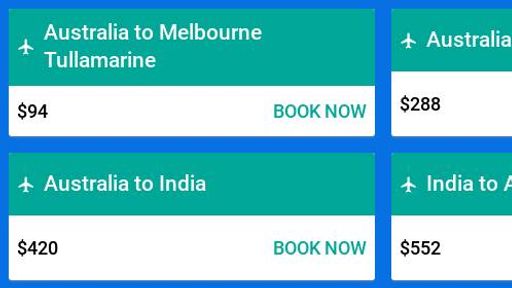This image appears to be a screenshot of a webpage, likely from Google Flights or a similar airfare comparison tool, showcasing flight options originating from Australia. The background has a medium blue hue with each flight option presented in individual boxes.

In the first row, the initial box on the left features a teal banner at the top. Within the banner, white text displays "Australia to Melbourne to La Marine," accompanied by a flight icon. Below this, the white section of the box lists a fare of "$94" and has a "Book Now" button in teal text aligned to the right.

The adjacent box on the right is partially cut off, but it shows a flight from "Australia" costing "$288."

In the second row, the full visible box on the left shows a flight from "Australia to India" for "$420" with a "Book Now" button similar to the other complete boxes.

To the right of this is another partially obscured box that mentions a route from "India to A" with a listed fare of "$552."

All visible flight options feature a common theme: departures from Australia with varied destinations and prices, suggesting that this is likely an "Explore" page offering diverse travel deals without specific filtering criteria beyond the departure location.